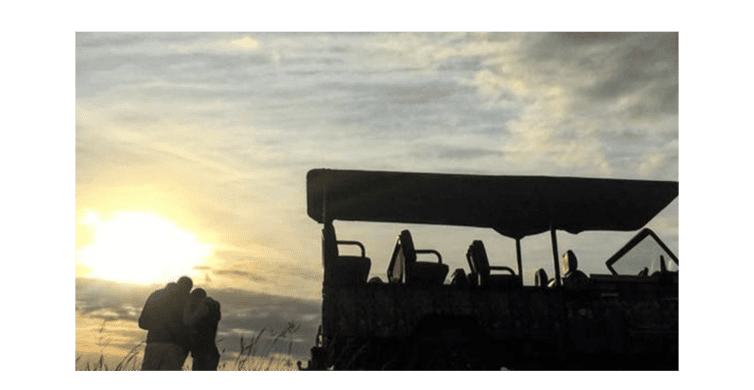In this entrancing sunset scene, a couple stands side by side, their backs to the camera, near a towering, silhouetted safari vehicle. The sky is a magnificent tapestry of blue and purple, accented by a setting sun that bathes the horizon in hues of yellow and rose. The couple appears to be holding onto each other, with the woman’s left arm wrapped around the man’s back, both seemingly engrossed in a map or phone in front of them. The safari vehicle, characterized by its four rows of seating and protective canopy, suggests an adventurous backdrop, shrouded in shadow due to the breathtaking yet dim twilight. The lower right corner displays a distinct silhouette of the vehicle, adding to the mystique of this picturesque African landscape, complete with wisps of clouds and tall grasses swaying in the gentle evening breeze.